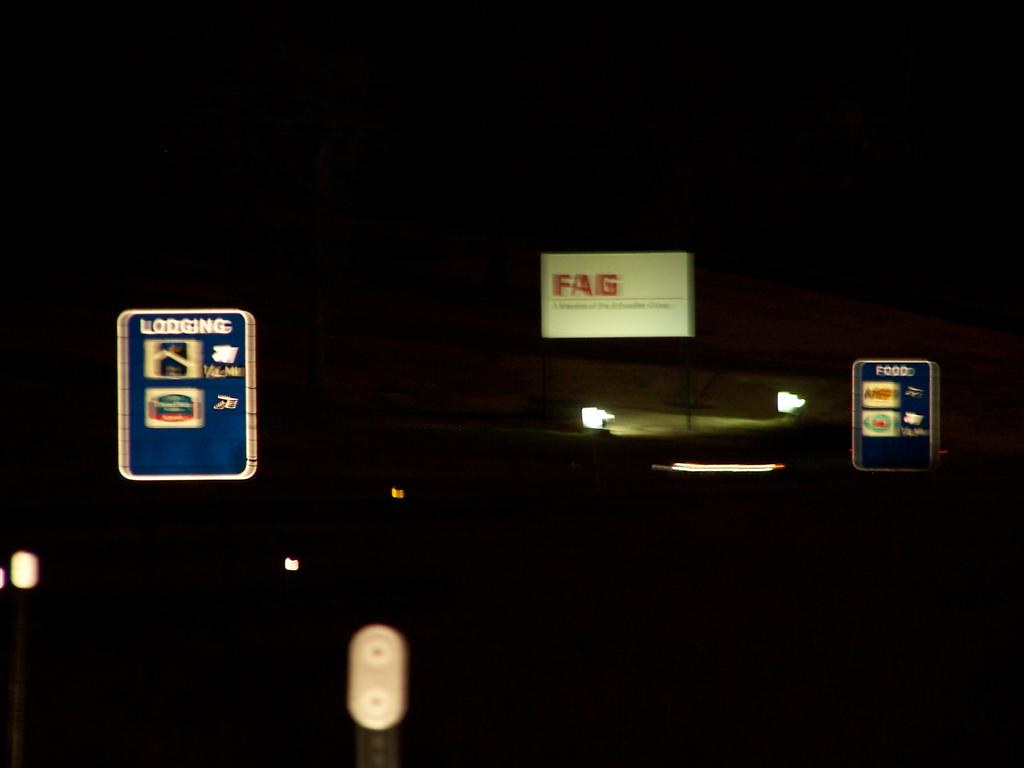Captured at night, this photograph showcases the eerie tranquility of a dark highway illuminated only by distant signage. Three large signs dominate the image against the pitch-black background. On the left, a blurred blue rectangular sign with reflective lining reads "Lodging," likely indicating nearby hotels. The reflective surface ensures the sign remains visible despite the blurry motion in the photo. In the center, a white billboard displays the bold red letters "F A G," with additional black writing underneath, although the distance obscures the smaller text. This sign is brightly lit, standing out clearly against the night sky. To the right, another blue rectangular sign mirrors the 'Lodging' sign's design but instead reads "Food," suggesting available dining options. The slight blur and angle of the photo hint that it was probably taken by someone driving down the highway, capturing these illuminated beacons from the window of a moving vehicle.